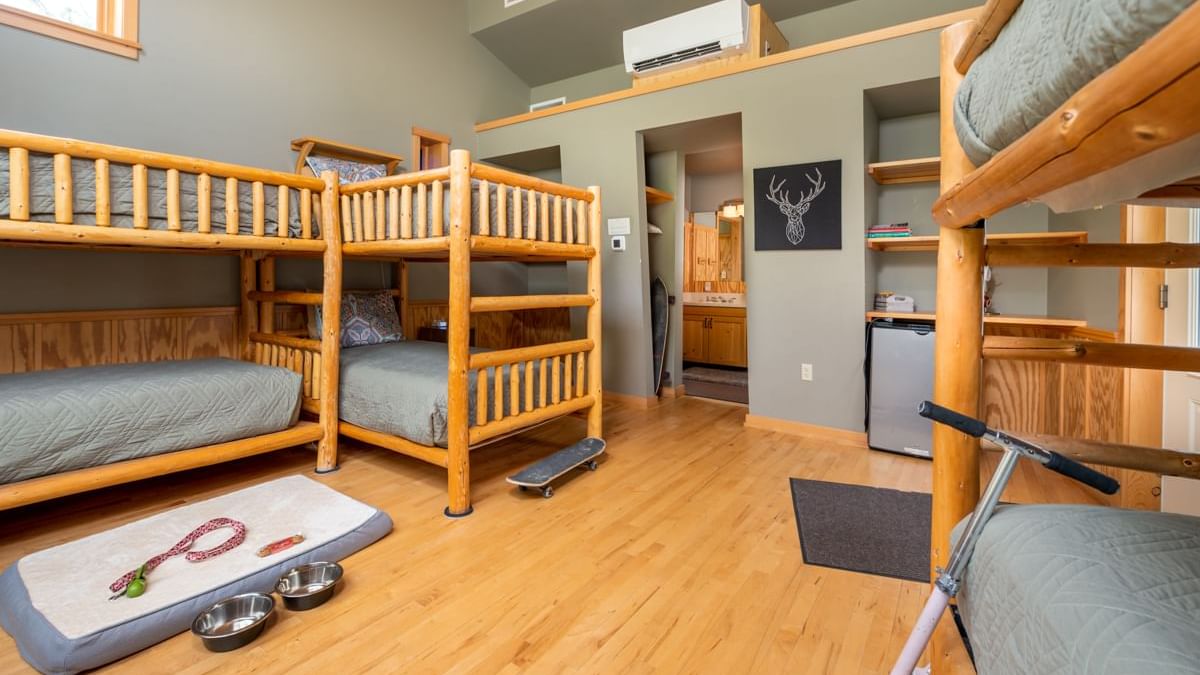This photograph showcases a rustic bedroom, likely in a lodge or cabin, furnished with three sets of full-size bunk beds made from log wood, emphasizing a farmhouse aesthetic. The bunk beds are arranged with one parallel to the wall and the others positioned at various angles, each adorned with gray blankets and patterned pillows. The room features hardwood or laminate flooring, upon which a skateboard and a scooter’s handlebars are visible, suggesting an active, youthful presence. 

A dog bed with a leash, rope toy, and two stainless steel pet bowls is located in the bottom left corner, indicating the presence of pets. On the floor, there is also a white mat with a blue border and two metallic pet balls. The walls are painted in a grey or grey-green hue, enhancing the cozy and modern ambiance. 

Above the mini bar fridge and three wooden shelves, a geometrically patterned deer picture adds a decorative touch. The air conditioning unit is situated above the door, which leads to an en suite bathroom with a cabinet matching the light tan wood theme. A grey carpet aligns in front of the door, further adding to the room’s warmth and homeliness. The photograph, taken at an angle, brightly lit, captures the inviting and multifunctional nature of this vacation home bedroom.